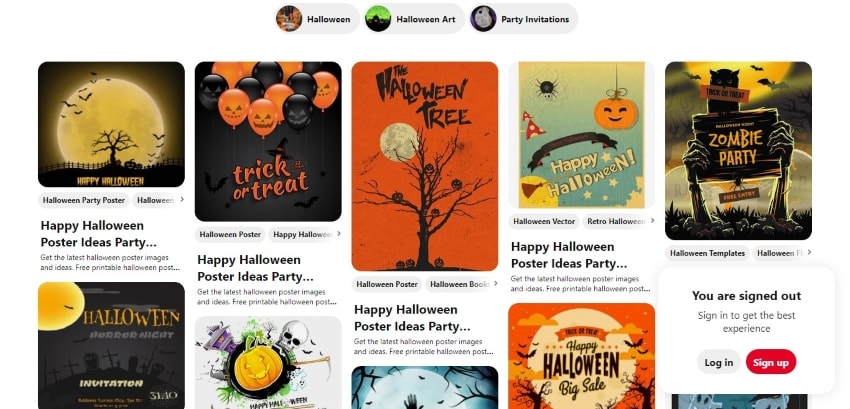This is a screenshot of a Pinterest-like application where a Halloween-related search has been performed. At the top of the screen, there are three oval-shaped headers, each accompanied by a small image. The first header on the left, labeled "Halloween," features a tiny black and orange picture. The central header, "Halloween art," displays a black background with a lime green image. The rightmost header reads "Party invitations," with a black background and a white shape.

Beneath these headers are five images in a row, each clickable and linked to more content. 

- The first image on the left captioned "Halloween party poster" depicts a night scene with a moon, a graveyard, and bats.
- Next is "Halloween poster, Happy Halloween," showcasing black and orange balloons with the text "Trick or Treat."
- The central image, titled "The Halloween tree," features a spooky tree under a moonlit sky, jack-o'-lanterns scattered on the ground and atop the tree.
- The image to the right, labeled "Happy Halloween, Halloween vector, or retro Halloween," has a blue background with various Halloween elements like spiders, jack-o'-lanterns, a moon, and a witch's broom.
- The final image on the right, "Zombie party as a Halloween template," presents zombie hands emerging from the ground, holding a sign with an owl on top that reads "Trick or Treat" and "Zombie Party."

Directly below this collection, there's a message indicating that the user is signed out with a prompt to sign in for the best experience. A grey "Login" button and a red "Sign Up" button are provided. Below this section, the tops of five more images are visible, though the details of these headers are not clearly seen.